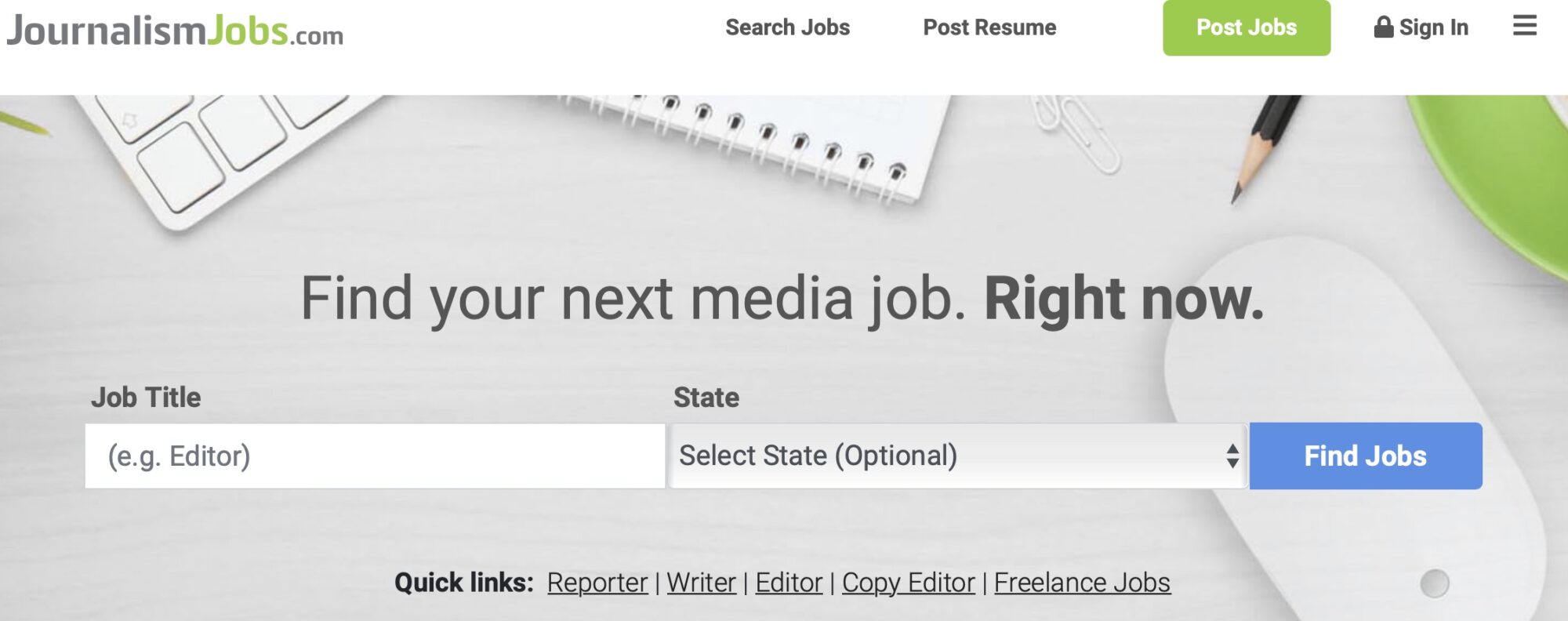**Caption:**

The screenshot captures the homepage of the "journalismjobs.com" website, featuring a white header at the top. On the left side of this header, the website's title is prominently displayed in a combination of gray and light green: "Journalism" and ".com" are in gray, while "Jobs" is in light green. To the right of the title, there is some negative space, followed by two gray sections labeled "Search Jobs" and "Post Resume."

Further to the right, after another section of negative space, a bright green button with white text stands out, reading "Post Jobs." To the right of this button, within the white header background, a gray lock icon is followed by gray text that says "Sign In," and next to it, three horizontal gray lines are stacked vertically, indicating a menu.

Below the header, a photograph showcasing a collection of objects creates a visually appealing composition. In the top left corner of the photo, a white keyboard is angled artfully. To its right, a white notebook is positioned at an opposite angle. Moving further right, two white paperclips are situated next to the tip of a mostly black pencil. Adjacent to the pencil is the corner of a green dish, with a white mouse positioned below it. 

Overlaying this photograph in the center, gray text reads: "Find your next media job right now," with the words "right now" in bold for emphasis.

Beneath this section, there are several elements designed for job searching. On the left, a white text box contains gray text in parentheses, "e.g., editor." Above this text box, dark gray bold text labels it as "Job Title." Next to it, to the right, another text box labeled "State" is presented with a light gray to white gradient background and gray text that says "Select state (optional)." Finally, a blue button with white text reading "Find Jobs" is positioned to the far right of this section, inviting users to initiate their job search.